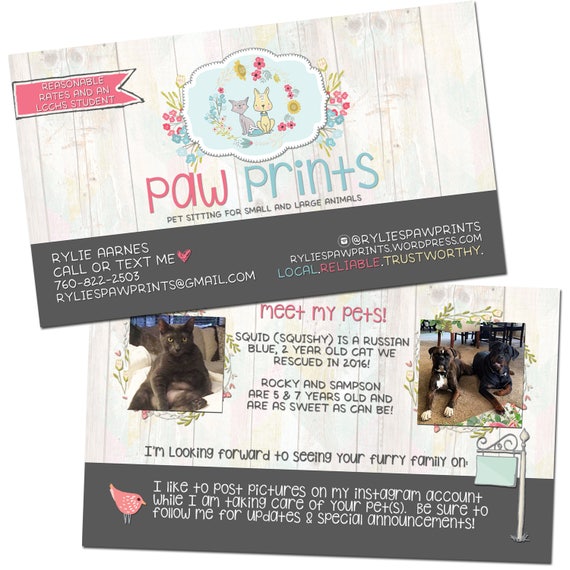**Detailed Caption for Pet Sitting Service Advertisement:**

This is an advertisement for a pet sitting service, suitable for various mediums including websites, magazines, or store window displays. The design comprises two vertically oriented, rectangular images featuring a soft pastel floral wallpaper and a brown footer along the bottom.

**Top Image:**
- **Background:** Pale-colored wallpaper adorned with light pastel flowers.
- **Main Visual:** At the center of the top image is a cloud-shaped design with a blue background, showcasing a gray cat and a tan dog surrounded by a garland of flowers.
- **Banner:** Positioned in the top left corner is a ribbon-style banner, outlined in black with a red center. The banner reads "Reasonable Rates" in white letters, with "an LCCHS student" written below.
- **Typography:**
  - Beneath the central cloud image, the words "Paw" (in red) and "Prince" (in blue) are prominently displayed. 
  - Below this, the text reads "Pet Sitting for Small and Large Animals" in black.
- **Contact Information:** Within the brown footer at the bottom:
  - Left side: The pet sitter's name, phone number, and email address.
  - Right side: Their Instagram handle and WordPress website.
  - Additional attributes in the footer: Words "Local" (in blue), "Reliable" (in red), and "Trustworthy" (in white).

**Bottom Image:**
- **Background:** Identical pastel floral wallpaper.
- **Visual Elements:** 
  - Upper left corner: A square image of a black cat.
  - Right-hand side: A square image featuring two young dogs.
- **Text:**
  - Across the center in red: "Meet My Pets".
  - Below in black: 
    - "Squid: Squishy as a Russian Blue, a two-year-old cat we rescued in 2016."
    - "Rocky and Samson: Five and seven years old, and as sweet as can be."
  - Further down, it reads: "I’m looking forward to seeing your furry family on."
- **Additional Features:**
  - To the right, a cartoon-style signpost with blank Post-it notes, where customers can add their own dates.
  - A notification in white text: "I like to post pictures on my Instagram account while I am taking care of your pets. Be sure to follow me for updates and special announcements." 
  - An illustration of a small red bird next to the white text.

This comprehensive advertisement encapsulates the essence of personalized and caring pet sitting services, highlighting reliability and a love for animals, augmented with vibrant visual and textual elements.